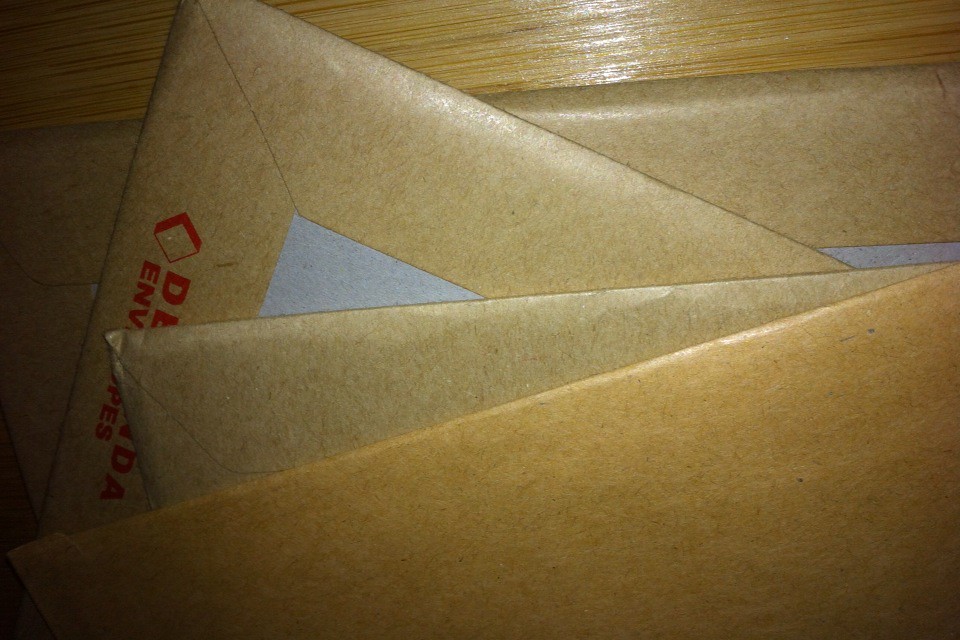The image depicts a close-up, slightly blurry photograph taken with a flash from above, showcasing four brown craft envelopes fanned out over a polished brown wooden table. The envelopes are arranged in a diagonal pattern, each partially obscuring the one beneath it. The top edges of the envelopes catch the light, reflecting the table's laminate shine. Two envelopes are facing up and two are facing down. The top envelope is plain brown, while the second reveals a hint of a red logo, only partially visible. The middle envelopes feature a distinctive white center framed by their brown cardboard borders. The bottom envelope, like the top one, appears simpler in design, emphasizing the fanned arrangement and the overall gradient of brown hues. Red text on the top or middle envelopes, likely part of the manufacturer’s logo—a 3D square diamond shape—is partially legible but mostly obscured. The photograph captures the textures and shades of the envelopes and their wooden backdrop in detail despite the image's low quality.